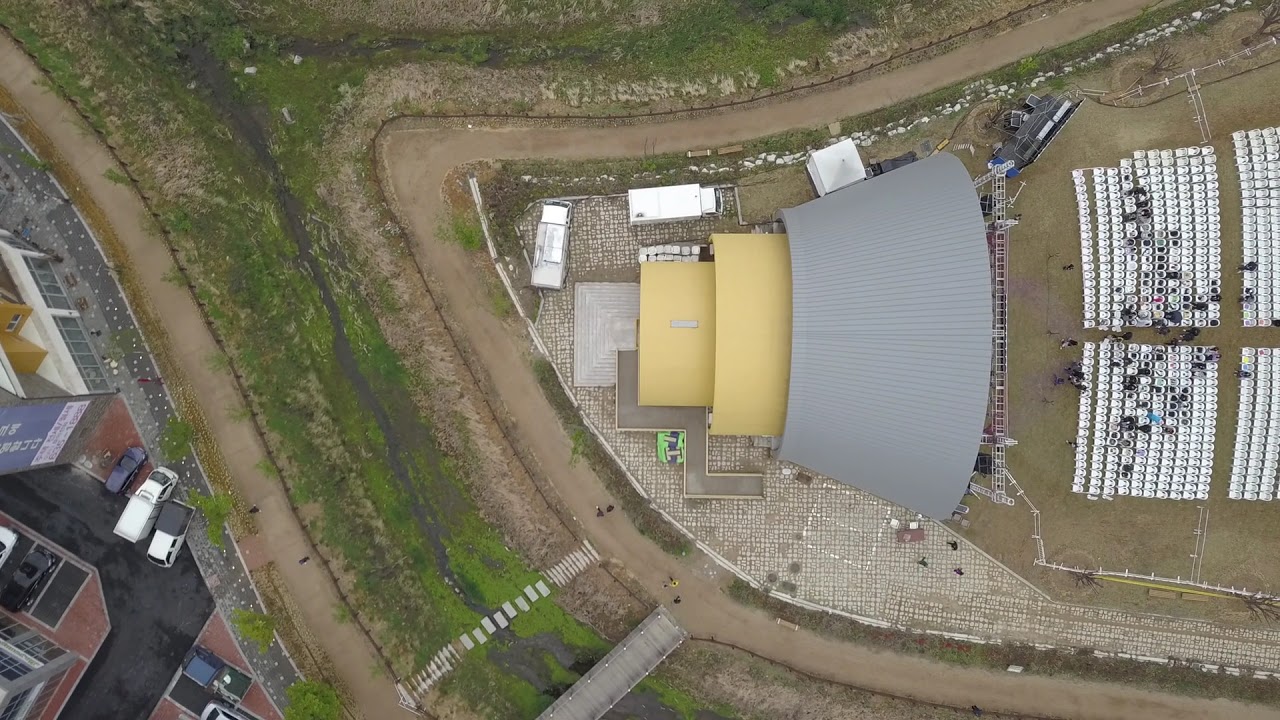This detailed aerial shot captures an expansive outdoor amphitheater with a distinctive yellow dome, reminiscent of a camera lens, framed by a blue outer edge. Positioned prominently in the center, the dome is surrounded to its right by hundreds of neatly arranged white lawn chairs, divided into four distinct sections, though the rightmost group is partially cropped out of the image. Directly left of the dome, a brick path crosses what resembles a damp area, indicating potential water flow, akin to a dam or water channel.

Encircling the amphitheater is a clearly visible road, flanked by green grassy patches and another parallel dirt road. Behind the seating area, there are multiple walkways with people meandering, evoking a sense of an event in progress. In the background, numerous white storage sheds are faintly visible.

Beyond this primary setup, the amphitheater is enveloped by a broader urban landscape, featuring buildings, houses, and parked cars, specifically noted in a parking lot situated in the lower left-hand corner of the frame. The bustling environment outside the theater, combined with detailed seating and architectural elements, paints a vivid picture of this lively, multifaceted venue.